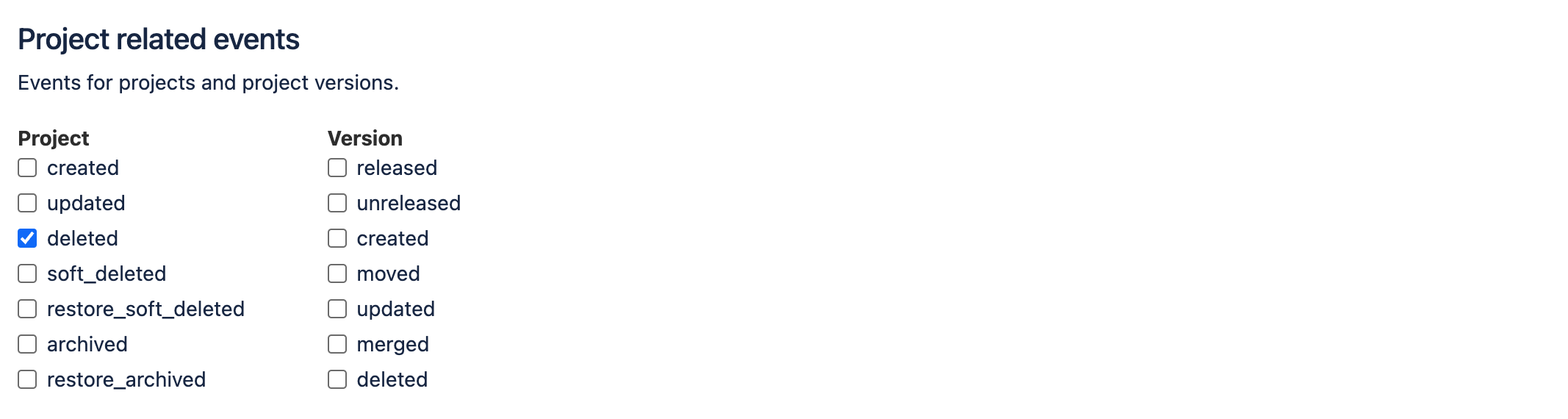The image depicts a clean and straightforward interface focused on project-related events. At the top, the heading reads "Events for Projects and Project Versions." Below this, the layout is divided into two main columns: "Project" on the left and "Version" on the right.

In the "Project" column, users can select various event options such as Created, Updated, and Deleted, with the "Deleted" option already checked and highlighted in blue, while the other options remain in white. Additional options include Soft_Deleted, Restore_Soft_Deleted, Archived, and Restore_Archived.

In the "Version" column, the selectable events include Released, Unreleased, Created, Moved, Updated, Merged, and Deleted.

The overall design is minimalistic, with no discernible indicators of the platform it appears on, such as phone icons or computer-specific elements. The image does not reveal any company affiliations or logos, leaving the origin and context of this interface unspecified.